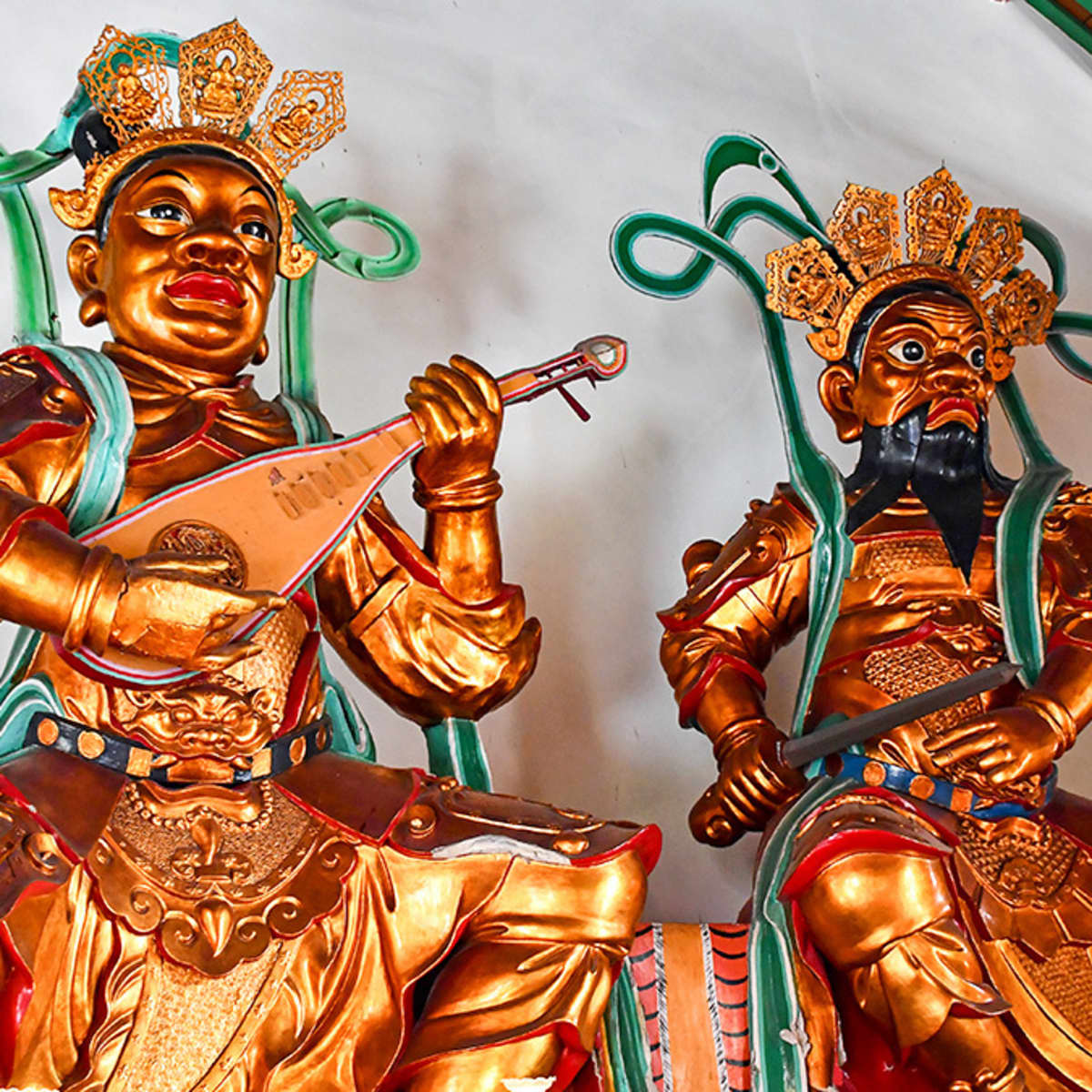The image showcases two intricately detailed bronze statues, posed against a white wall adorned with green lines and symbols that create an optical illusion of green straps draping over their shoulders. Both statues are predominantly bronze in color, with distinct black eyes and red lips, and they cast noticeable shadows on the wall behind them. 

The statue on the left, identified as a queen, features dark-colored hair and is clean-shaven. She wears a bronze crown with three pentagon-like petals, has a belt with a prominent gold plate over the waist area adorned with round blue circles, and green straps cascading over her shoulders. Her right hand strums a metallic ukulele or similar string instrument while her left hand grips the handle. She appears to be seated, with her left leg bent at the knee, partially obscured.

To her right stands the statue of a king, distinguished by a black beard and a crown with five pentagon-like petals. He grips a long sword in his right hand, pointing it outward from his hip. Like the queen, the king also has green straps over his shoulders, adding to the optical illusion with the wall behind them. He sports a blue belt with orange circles and has bronze armor with what appears to be a protective piece or shield across his right knee. Both statues are seated on what seems to be green-colored thrones, evidenced by the green backdrop, although the base is not visible.

These regal statues, with their detailed adornments and the interplay of colors, textures, and positioning, create an evocative scene, juxtaposing royal elegance with artistic optical illusions.